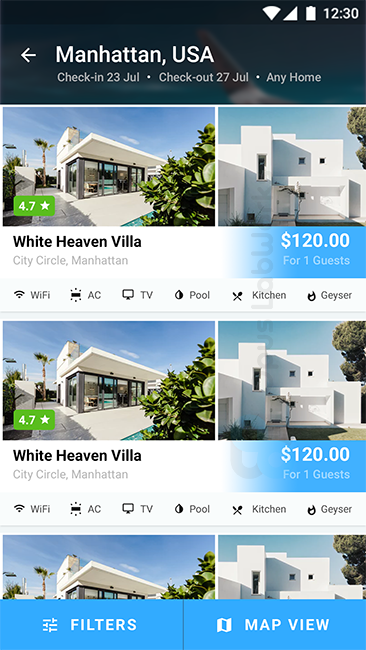A dimly lit smartphone screen displays a booking application on a dark blue-gray background. The top left corner features a battery icon, full signal strength for Wi-Fi, cellular data bars, and a clock displaying 12:30, all in white. Below, there is a navigation arrow pointing left, alongside text that reads "Manhattan, USA" with check-in on 23 July and check-out on 27 July.

The main content showcases three hotel options under the heading "any home." The first option is "White Heaven Villa," depicted with two images of modern, blocky, white buildings. The hotel has a rating of 4.7 stars, highlighted in a green box. Beneath the images, the name "White Heaven Villa" appears again, alongside "City Circle, Manhattan." The price is listed at $120 for one guest. The amenities include Wi-Fi, AC, pool, TV, kitchen, and a geyser.

The second option mirrors the first, with identical images and a matching 4.7-star rating in the same green box. Similarly, it is also named "White Haven Villa," priced at $120 for one guest, noted in blue text under the price.